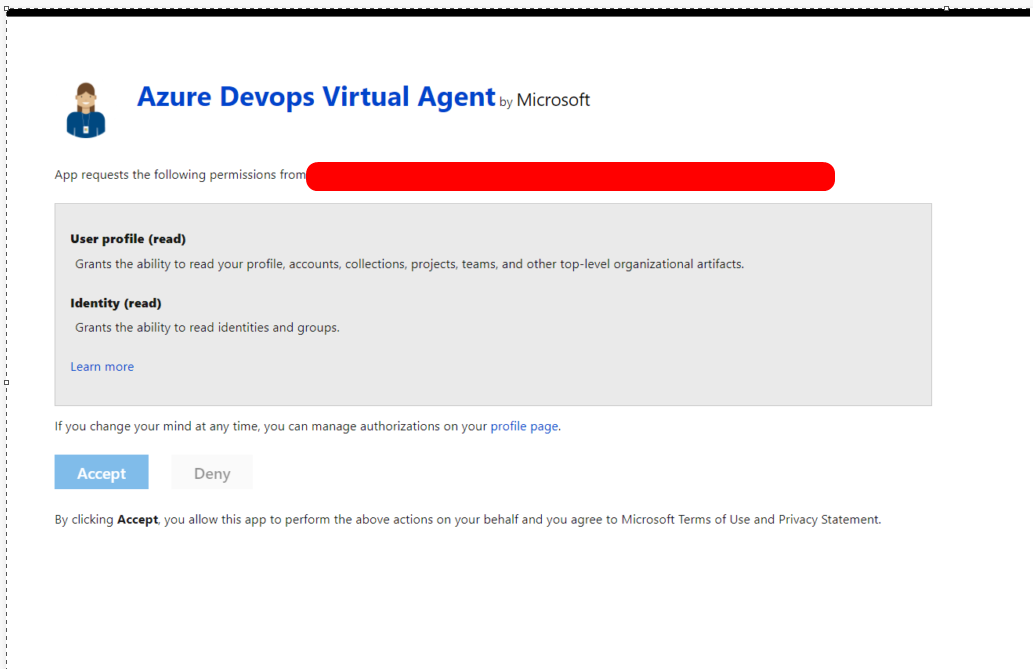This screenshot captures an incomplete image cropping operation on a desktop, evidenced by the visible dotted line partially encircling part of it. The cropped section reveals a black bar at the top, followed by a cartoon depiction of a woman with brown hair, donning a blue sweater and an ID badge. Below the illustration, text reads: "Azure DevOps Virtual Agent by Microsoft."

The image continues with the phrase "App requests the following permissions from," although the rest of the sentence is obscured by a red rectangle, concealing crucial details. Visible permissions include "User profile, read," in bold, with subsequent explanatory text: "Grants the ability to read your profile, accounts, collections, projects, teams, and other top-level organizational artifacts."

Further listed is "Identity, read," also in bold, accompanied by, "Grants the ability to read identities and groups." Below this section is a blue button labeled "Learn More." Additional guidance appears, stating: "If you change your mind at any time, you can manage authorizations on your profile page," linked to the appropriate profile management section.

The options to "Accept" or "Deny" the permissions are present but currently grayed out. A concluding note explains: "By clicking accept, you allow this app to perform the above actions on your behalf and you agree to Microsoft terms of use and privacy statements."